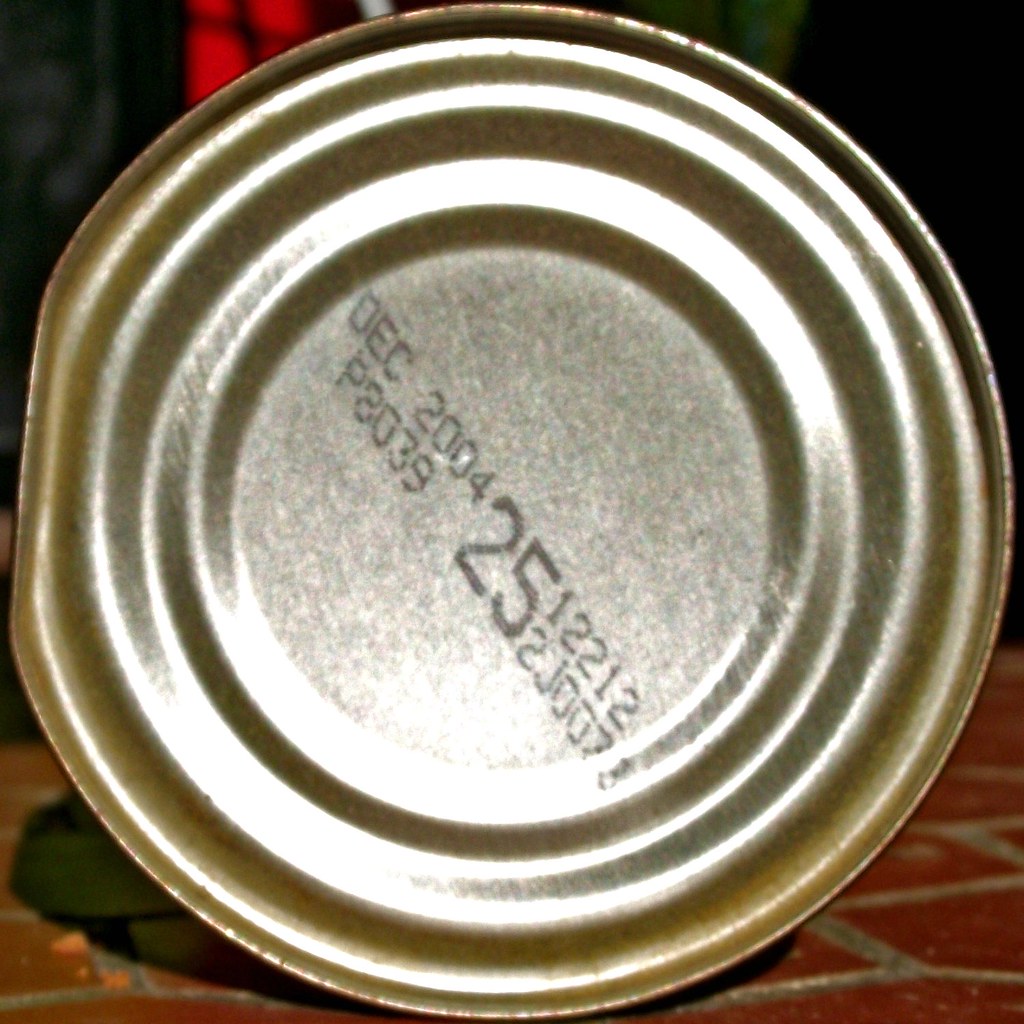The image prominently features the bottom of a canned good with various markings. The silver base of the can is labeled with diagonal text reading "December 2004 P8039" and a large "25" positioned centrally. Further right, the numbers "12212" appear with a backwards "S" just above "J007." The can's bottom surface is slightly dented on the left side, emphasizing its worn condition. The background is a blurred mix of black and red hues, suggesting a tile or possibly a red brick surface with gray mortar. The can takes up most of the frame, indicating it was likely photographed using an older camera, resulting in a grainy and less detailed image compared to modern standards. The setting is indistinct but suggests a rustic or perhaps industrial environment.